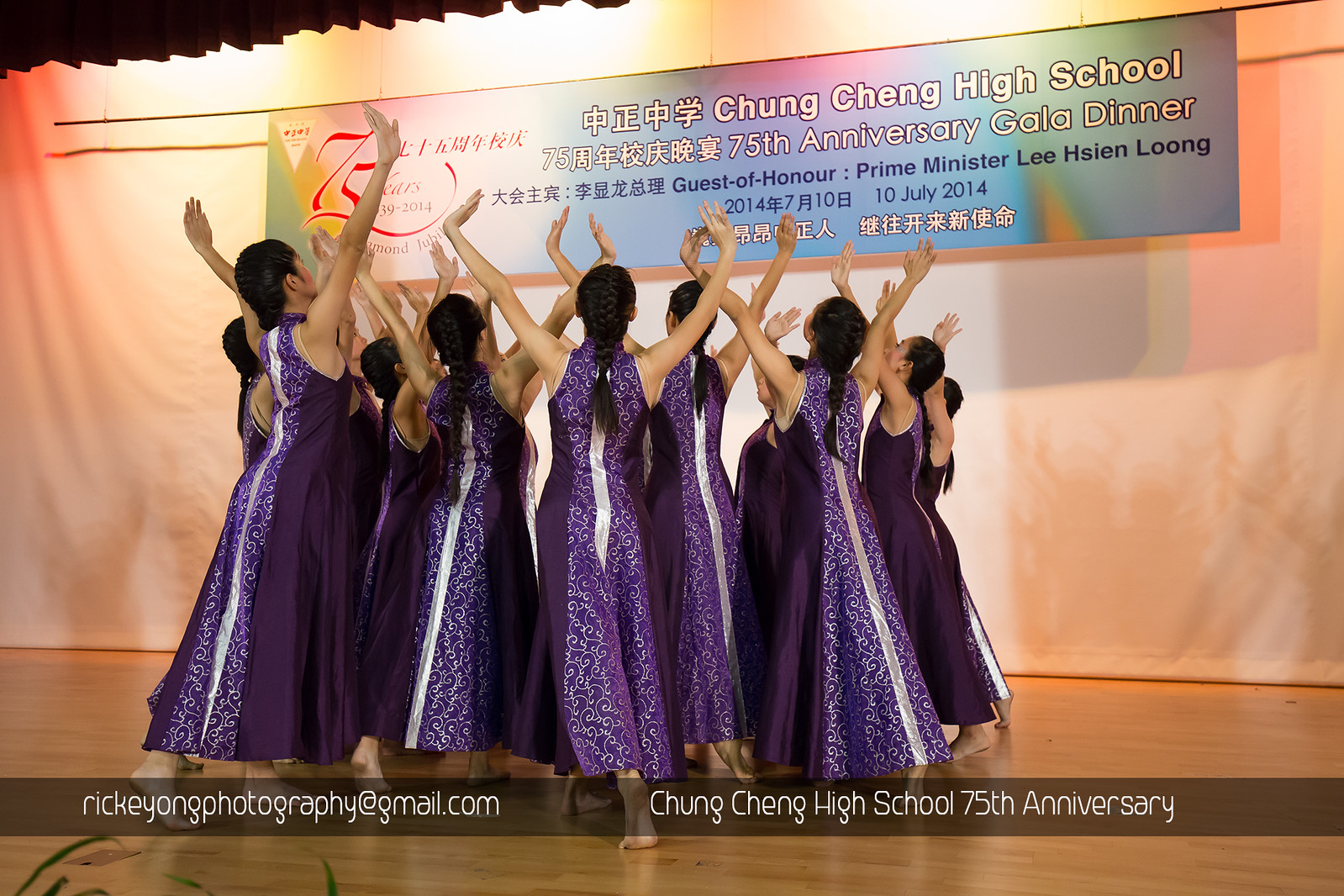This color photograph captures a school dance performance on a stage. A small group of women, all with long black hair, are dressed in identical long gowns that are purple with silver designs, extending to the floor and concealing their bare feet. They are facing away from the camera with their arms gracefully outstretched upwards. The scene is set before a dual-language banner in English and Chinese, which reads: "Cheung Chang High School 75th Anniversary Gala Dinner. Guest of Honor Prime Minister Lee Hsien Loong, 10 July 2014."